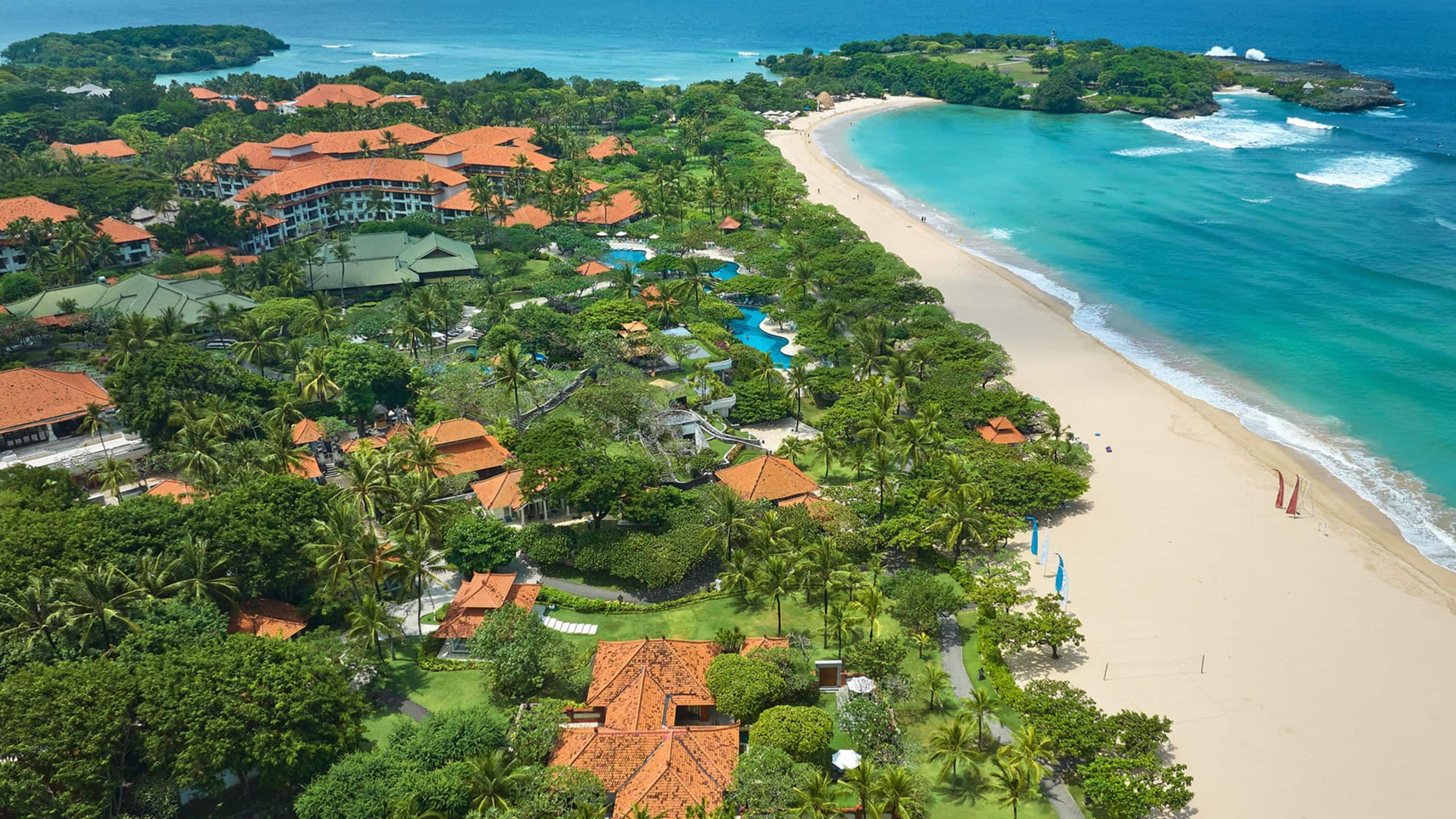This detailed aerial photograph captures a picturesque resort located on a tropical island, possibly in Bali or the Caribbean. The image prominently showcases a beautiful beach with white sand on the far right, where crystal-clear, vibrant green-blue waves gently break upon the shore. Flanking the beach, there are intriguing long structures in blue and red colors, which could either be flags or angular surfboards.

A lush, green peninsula juts out into the water on the top right, seamlessly connecting to the mainland adorned with abundant palm trees and verdant vegetation. The resort itself dominates the left-hand side of the image, featuring an array of white buildings crowned with red roofs, including what appears to be large three or four-story hotels and smaller structures likely used for various activities. 

Near the top of the image, there are several bright blue swimming pools, surrounded by cabanas and other amenities, indicative of the resort's extensive grounds. Further inland, interspersed among the trees, small buildings dot the landscape, adding to the idyllic charm. Another peninsula emerges in the top left, and surrounding both peninsulas and the island is expansive, tranquil water that extends beyond the frame, emphasizing the secluded and serene nature of this tropical paradise. The absence of the sky in the photograph keeps the focus trained on the luxuriant greenery, resort amenities, and the pristine beach that seamlessly melds with the encompassing waters.